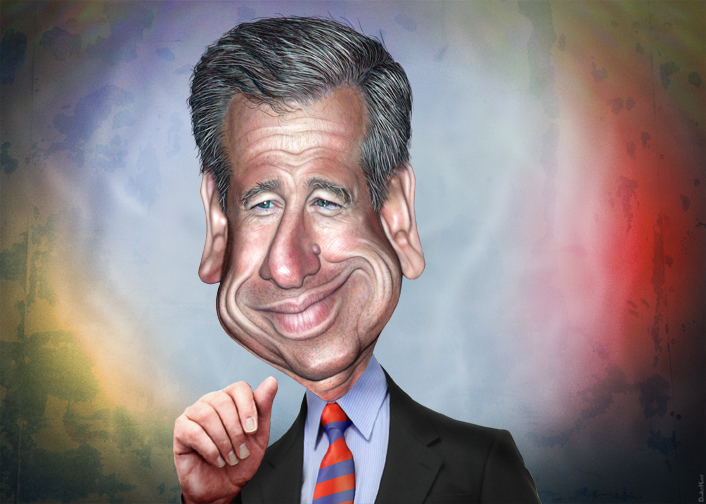The image is a detailed caricature of a white male politician, with exaggerated facial features such as a large nose, cheeks, and ears, giving it a distinct comic strip appearance. He has salt-and-pepper hair that appears gray, silver, and white. He is smiling widely and has a distinctive mole on his nose. The man is dressed in a gray suit, a blue shirt, and a red and blue striped tie. His right hand is raised with the fingers folded down, as if waving. The colorful, swirling background includes shades of black, white, gray, red, light blue, dark blue, medium blue, pink, yellow, peach, and purple, which create a dynamic and somewhat chaotic visual effect.